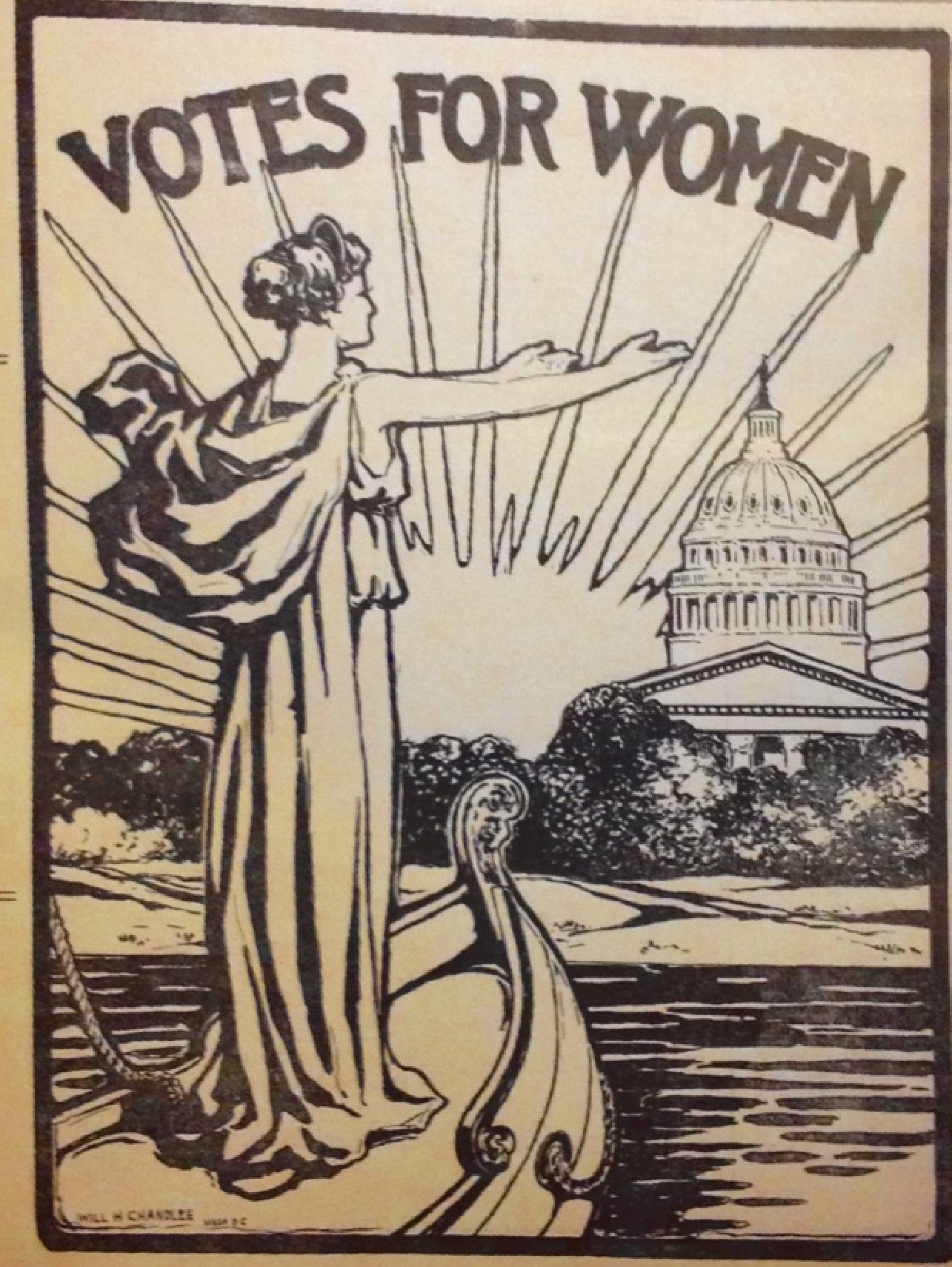This black and white suffragette poster has an old-time feel and appears somewhat yellowed with age. Framed by a black border, it prominently features the bold, uppercase headline "Votes for Women" curved across the top. Below this, a striking image captures attention: a woman, styled as a Roman goddess in a toga with billowing robes and coiffed hair, stands at the bow of an ancient-style boat with an ornamental prow. Her outstretched arms reach towards the right side of the poster where the iconic dome of the U.S. Capitol building rises, partially obscured by the horizon. The boat is seen gliding on calm waters toward the shore, where a strip of vegetation marks the boundary. Behind this powerful scene, an outlined sunburst symbolizes the dawn of a new era. This poster vividly conveys the aspirations of the women's suffrage movement, with Lady Liberty guiding the way toward democratic inclusion and the extension of voting rights to women.